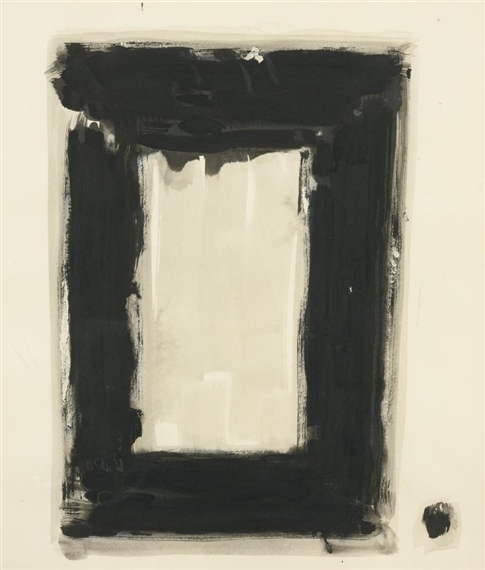The image showcases an abstract painting featuring a composition of rectangles and a dot on a very light yellow, almost cream-colored background. Central to the artwork is a vertically oriented, cream-colored rectangle that almost seamlessly blends with the background. A black rectangle frames this inner rectangle, forming a border around it. The brushstrokes are evident, with streaks and slight drips, indicating a rough, unsmoothed application of paint. This adds texture and depth, highlighting variances in the yellow and cream hues. In the bottom right corner, a black dot or smudge, resembling an incomplete fingerprint, disrupts the symmetry with its irregular edges. Overall, the painting exudes a crude yet intriguing abstract quality, with the central light rectangle creating a contrast against the encasing black shape and the subtle imperfections lending a raw, unfinished feel to the piece.